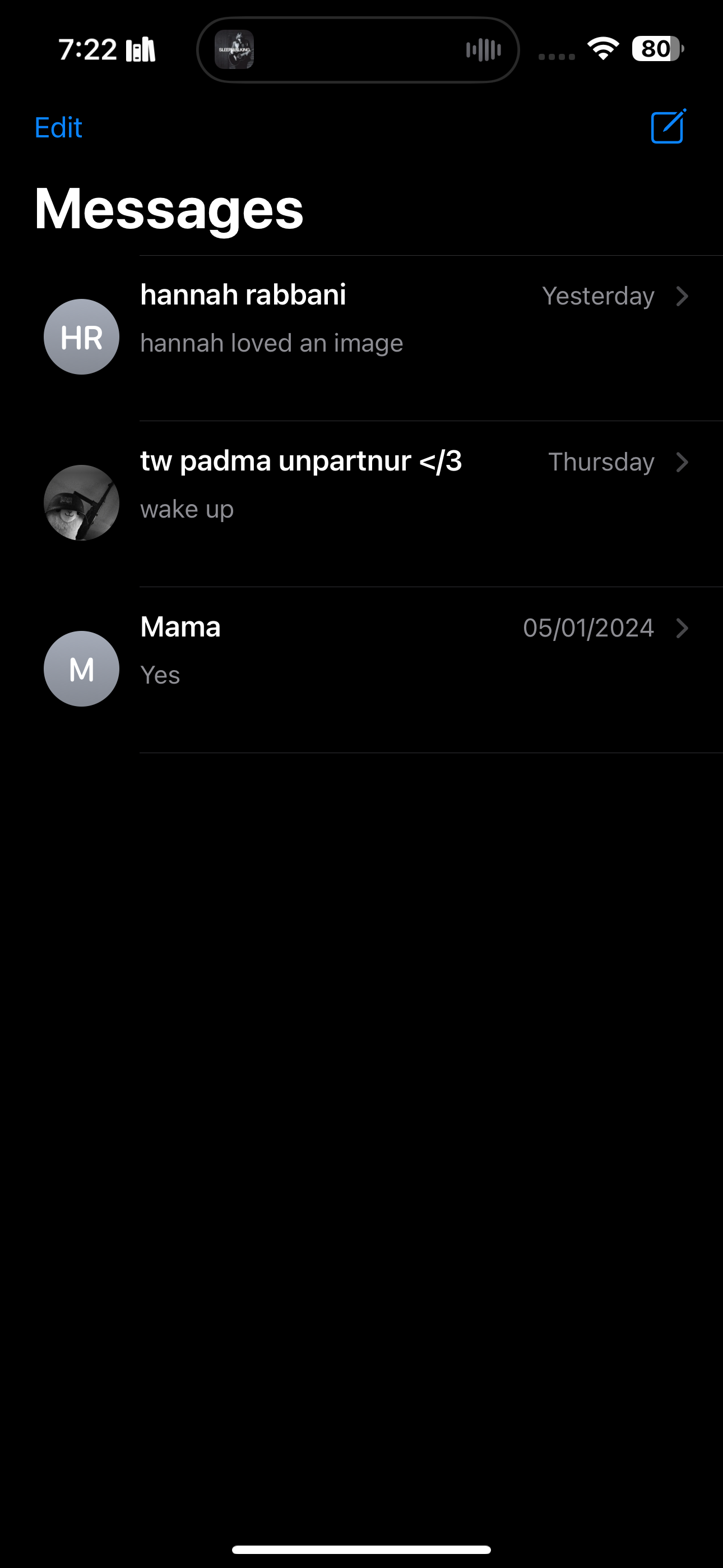This image is a screenshot of a messaging application displayed on a mobile phone. The screenshot begins with a black top bar on the left corner. Below this bar is a blue text reading "Edit" aligned to the left. On the far right, aligned with the header, there is a blue square icon with rounded corners featuring a blue pencil icon tilted at a 45-degree angle. 

Aligned to the left, just beneath this header section, there is white text that reads "Messages." Below "Messages," there are three distinct conversation entries, each separated by very thin, dark grey lines.

1. The first conversation features a light grey circle on the left with white text that reads "HR." To the right is the name "Hannah Rabbani," written in white text. Below this name, in small grey text, it states, "Hannah loved an image." To the right of this text, "Yesterday" can be seen with a rightward-pointing arrow next to it.

2. The second conversation displays a round profile picture featuring a black-and-white animal on the left. To the right of the picture is the name "TW Padma Unpartner" in white text, followed by a heart emoticon with a slash through it. Below the name, in grey text, it reads "Wake up." At the top right corner, it states "Thursday," accompanied by an arrow pointing to the right.

3. The third conversation shows a light grey circle on the left with a white "M" within it. To the right is the name "Mama," indicated in white text. Below this, in grey, it simply says "Yes." Above to the right, it shows the date "05-01-2024" with a rightward-pointing arrow.